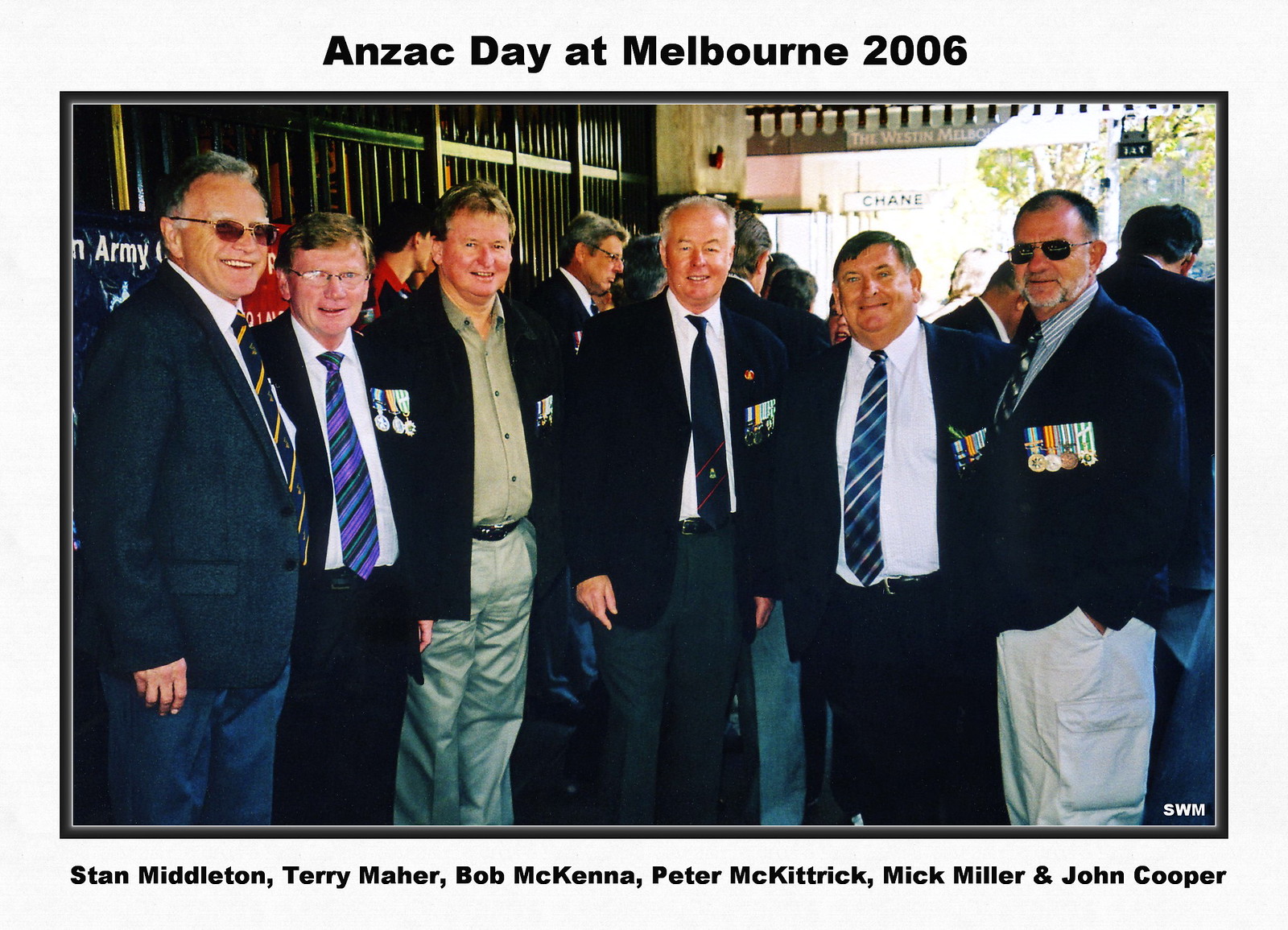This photograph depicts a gathering of six older white men, dressed in dark suits and collared shirts, with most of them wearing ties, standing on a sidewalk in front of a building. Their names, listed at the bottom of the photo, are Stan Middleton, Terry Maher, Bob McKenna, Peter McKittrick, Mick Miller, and John Cooper. Noteworthy details include John Cooper and Bob McKenna wearing aviator-style and rose-tinted glasses, respectively. All the men have short, graying, or balding hair. The group appears to be attending an ANZAC Day event in Melbourne in 2006, as indicated by a white border around the photo that bears this inscription. In the background, other men can be seen socializing, enhancing the reunion-like atmosphere. A sign on the building behind them includes the word "army," which aligns with the ANZAC Day theme. Most of the men are adorned with medals, suggesting their veteran status, and possibly their participation in the Australia and New Zealand Army Corps.